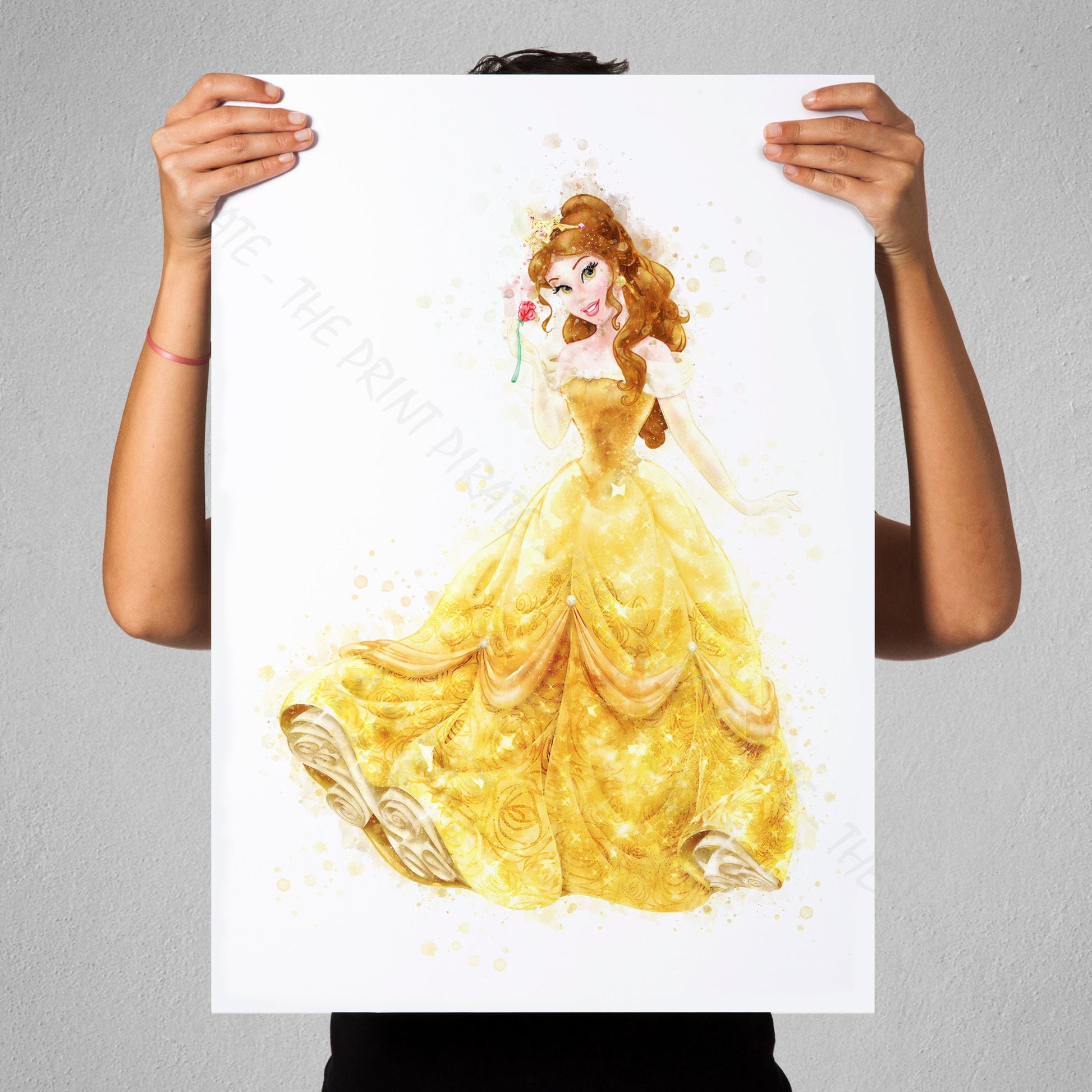In the image, a tanned individual holds up a rectangular, watercolored print of Belle from Disney's Beauty and the Beast against a plain white backdrop. The print, extending from the top of their head to their midsection, obscures their face, revealing only the top tufts of their dark brown hair and well-manicured hands. Belle, depicted in a modern, sparkly illustration, stands enrobed in her signature golden yellow ball gown, highlighted with shimmering sparkles. She has long, artfully curled hair adorned with a tiara and holds a delicate rose beside her. A watermark reading "Print Pirates" runs diagonally across the artwork. The person's right wrist sports a small pink rubber bracelet.